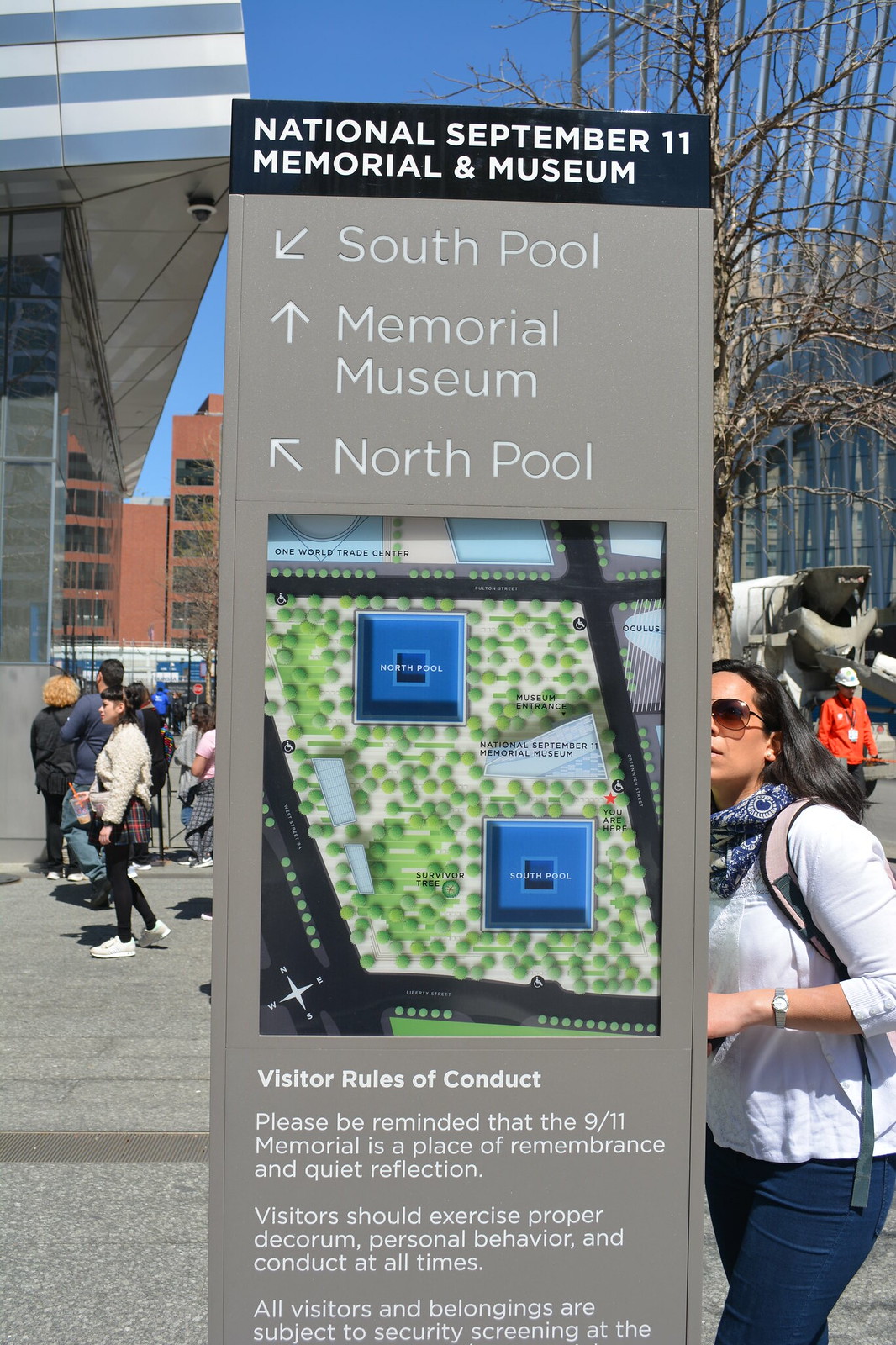The image depicts an outdoor area resembling a sidewalk or courtyard, where several people can be seen milling about. In the foreground, centrally positioned, stands a tall informational sign with a gray background. The top of the sign features a prominent black banner with the text "National September 11th Memorial and Museum." Below this header, there are arrows indicating the directions to key landmarks: "South Pool" pointing down left, "Memorial Museum" pointing straight ahead, and "North Pool" pointing up left. The central section of the sign showcases a detailed map illustrating the area where the World Trade Center once stood, now transformed into pools surrounded by lush vegetation. At the bottom of the sign, there is an advisory stating: "Visitors' Rules of Conduct: Please be reminded that the 9-11 Memorial is a place of remembrance and quiet reflection. Visitors should exercise proper decorum, personal behavior, and conduct at all times." A woman dressed in a white top and black pants, with a blue bandana and sunglasses, is seen actively looking at the sign. In the background, there are several buildings, including a glass structure with a roof featuring blue and white stripes, and a taller glass facade to the right. Further back, additional buildings with reddish exteriors and black windows can be observed against a strikingly blue sky, indicating a clear day.